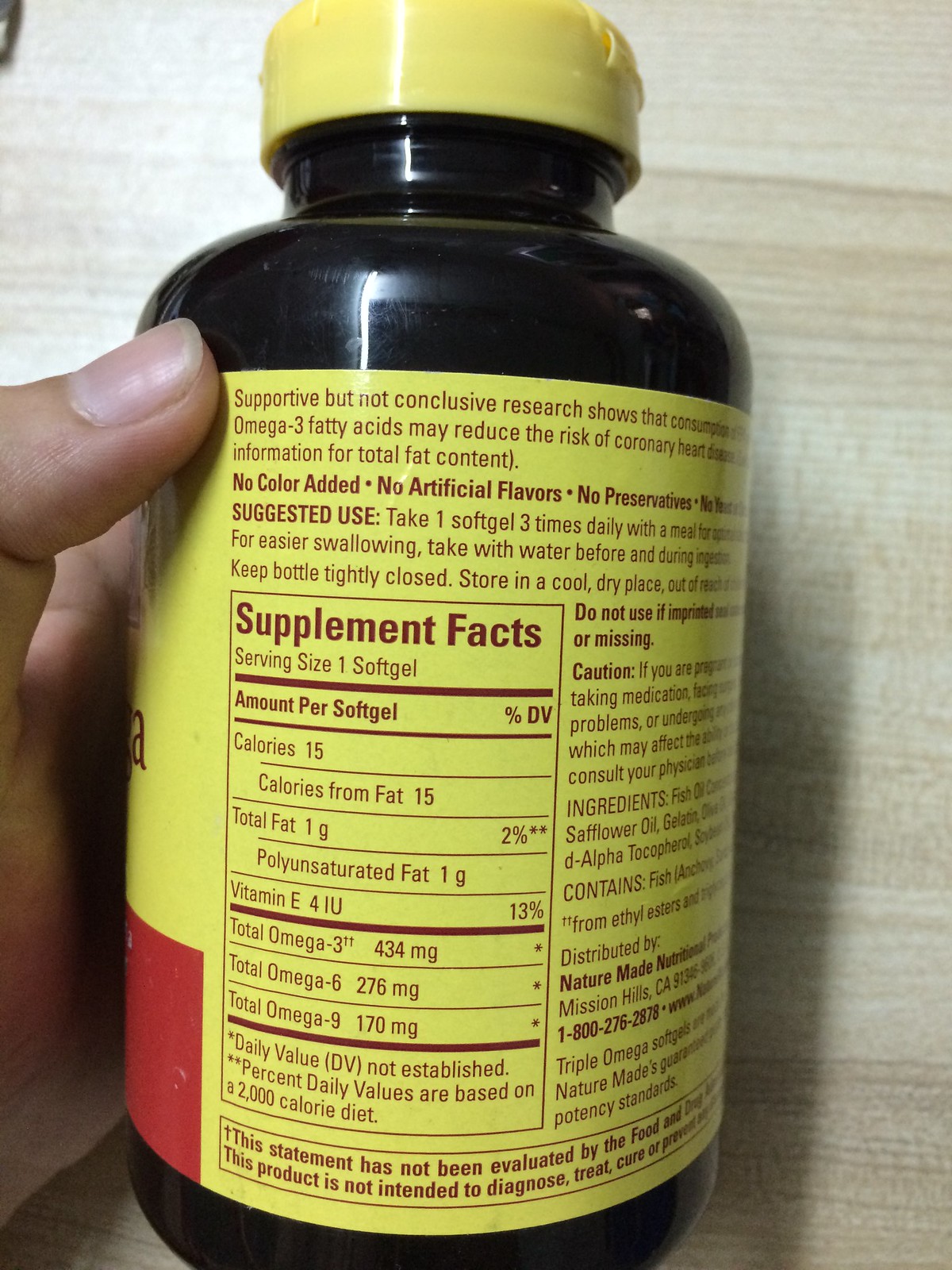The image displays a close-up view of a black plastic bottle with a yellow cap and a yellow label, held by a hand on the left side of the frame, showcasing the thumbnail and part of the hand with tan skin and white fingernails. The bottle features detailed nutritional and supplemental information in dark red text. The label specifies serving size as one soft gel, with nutritional details including 15 calories (all from fat), 1g of total fat, 1g of unsaturated fat, 4 IU of Vitamin E (13% DV), 134 mg of total Omega-3, 276 mg of total Omega-6, and 170 mg of total Omega-9. Additionally, the label includes warnings, usage instructions, and contact information for further inquiries. In the background, there's a light gray wooden surface. The text also indicates a partially readable statement about supportive research on the potential health benefits of Omega-3 fatty acids.